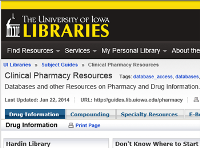This image captures a blurred screenshot of the University of Iowa Libraries website, particularly highlighting their Clinical Pharmacy Resources page. At the top of the webpage, there are four navigation tabs visible: "Find Resources," "Services," "My Personal Library," and the last tab which is partially cut off but likely reads "About." The main title on the page reads "Clinical Pharmacy Resources," followed by a subheading, "Databases and Other Resources on Pharmacy and Drug Information," indicating that the content is geared towards providing specialized resource information. The page appears to have been last updated on January 22, 2014. A segment labeled "Drug Information" is distinctly highlighted in blue, presumably denoting a clickable link or important resource category. The web address (URL) is visible in the middle part of the screen, although it is not legible in this blurry image. Additionally, three other resource categories are mentioned: "Drug Information," "Compounding," and "Specialty Resources." Furthermore, there is a reference to the Hardin Library, which may be part of the university library system. The overall layout appears congested, potentially leaving users unsure of where to begin their search.